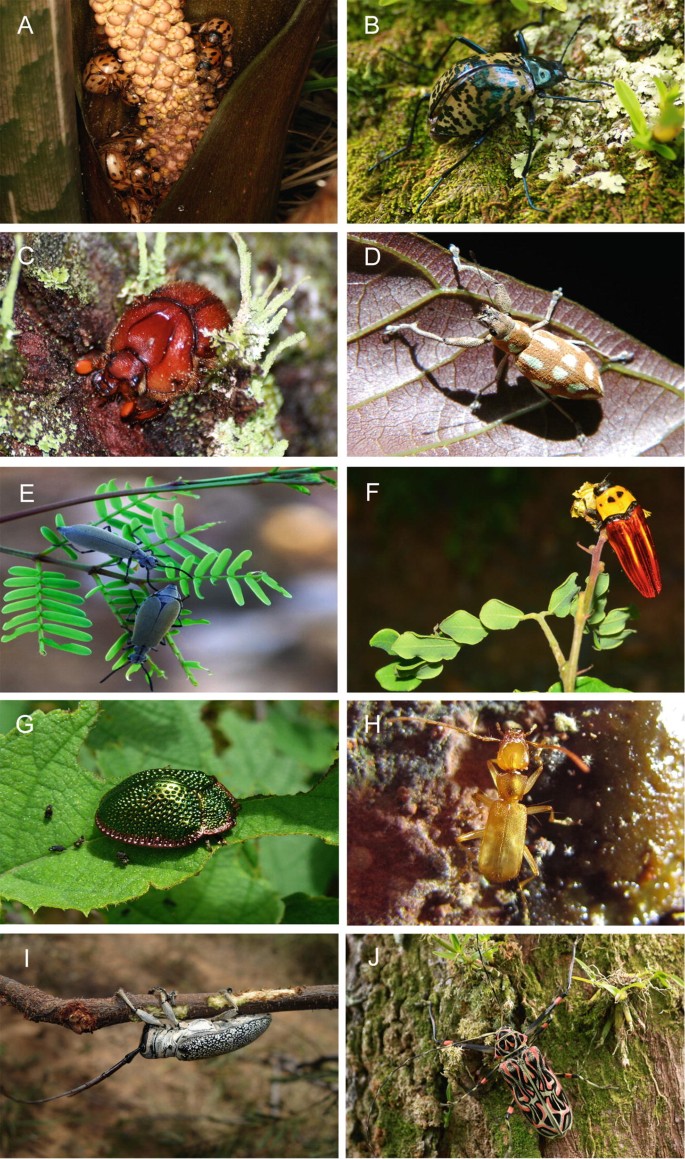The image is a compilation of ten vivid and colorful photographs showcasing various types of bugs and plant elements, labeled alphabetically from A to J in the top left of each picture. The photos are rich in greens, browns, reds, and blues, and seem to be presented in two vertical columns, potentially for a nature magazine or educational publication. 

In detail, Picture A shows a plant next to a moss-covered rock with a ladybug perched atop. Picture B features a beetle with a tiger-striped pattern on bark or moss. Picture C presents a bright red beetle on moss. Picture D depicts a light brown beetle with white polka dots on a leaf. Picture E shows two blue beetles on a fern frond. Picture F captures a red and yellow beetle on a plant. Picture G exhibits a small green beetle resembling an emerald hemisphere on a leaf. Picture H illustrates a golden yellow oblong beetle on bark. Picture I presents a silver beetle on a twig. Finally, Picture J shows what appears to be some fungus on moss-covered tree bark. Each image captures detailed views of the insects in their natural habitats, emphasizing both their unique colors and patterns.